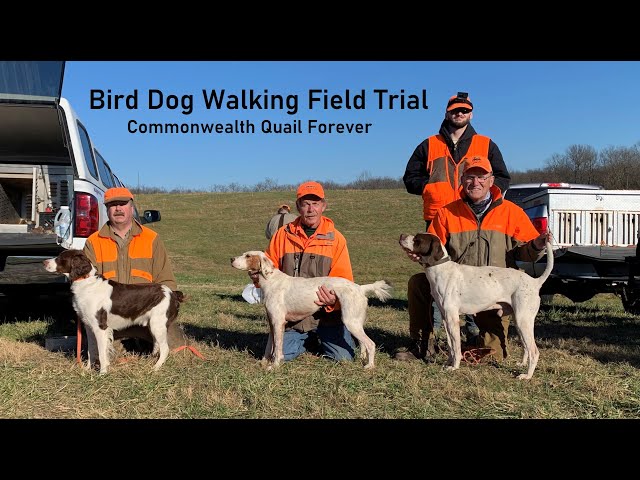In a sunlit field, four hunters clad in orange and brown hunting gear pose with their dogs for a commemorative photo. The vibrant blue sky casts a lively light on the scene, highlighting both the dead and living patches of grass. The centered text at the top reads "Bird Dog Walking Field Trial Commonwealth Quail Forever". The three hunters in the front are kneeling, each gently holding a distinct breed of hunting dog, all facing towards the left. They wear orange hats and coats accented with brown. Notably, two of the men sport mustaches. The fourth hunter stands in the background to the right, dressed similarly but with a vest over a black sweatshirt, and what appears to be a GoPro camera mounted on his hat. To the left of the scene is the open back of an SUV, while a trailer is visible on the right, framing the tableau of this organized hunting event.